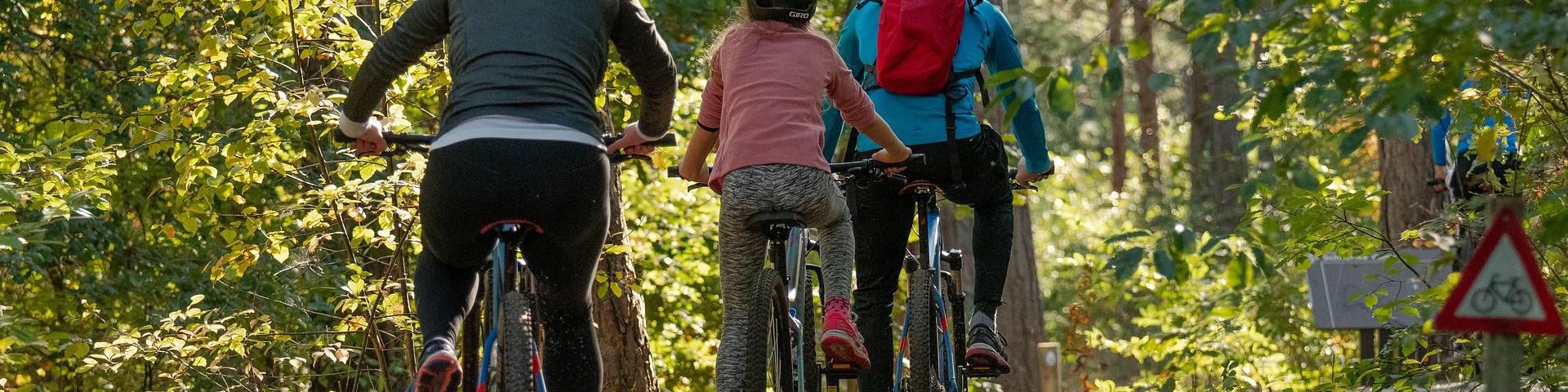The image captures a vibrant outdoor scene in a lush forest area, brimming with greenery and dense foliage. Three cyclists, viewed from behind, are riding away from the camera. The first biker, clad in a long-sleeve blue shirt, a red backpack, and black pants, leads the way. Positioned centrally is a young girl, wearing a helmet, a long-sleeve pink shirt pushed up to her elbows, black and white zebra print pants, and pink shoes. Following her is another adult, identifiable by her long-sleeve gray top over a white shirt and black pants. The path they are on is flanked by tall trees and verdant bushes. On the right side of the image, a red-bordered triangular sign with a white center depicting a bicycle serves as a warning of bike presence. Adjacent to it, partially obscured amidst the foliage, is a structure resembling a mailbox, and possibly a person dressed in blue, blending into the natural surroundings. The photo is rectangular in shape, providing a wide, detailed view of this serene and active moment in nature.